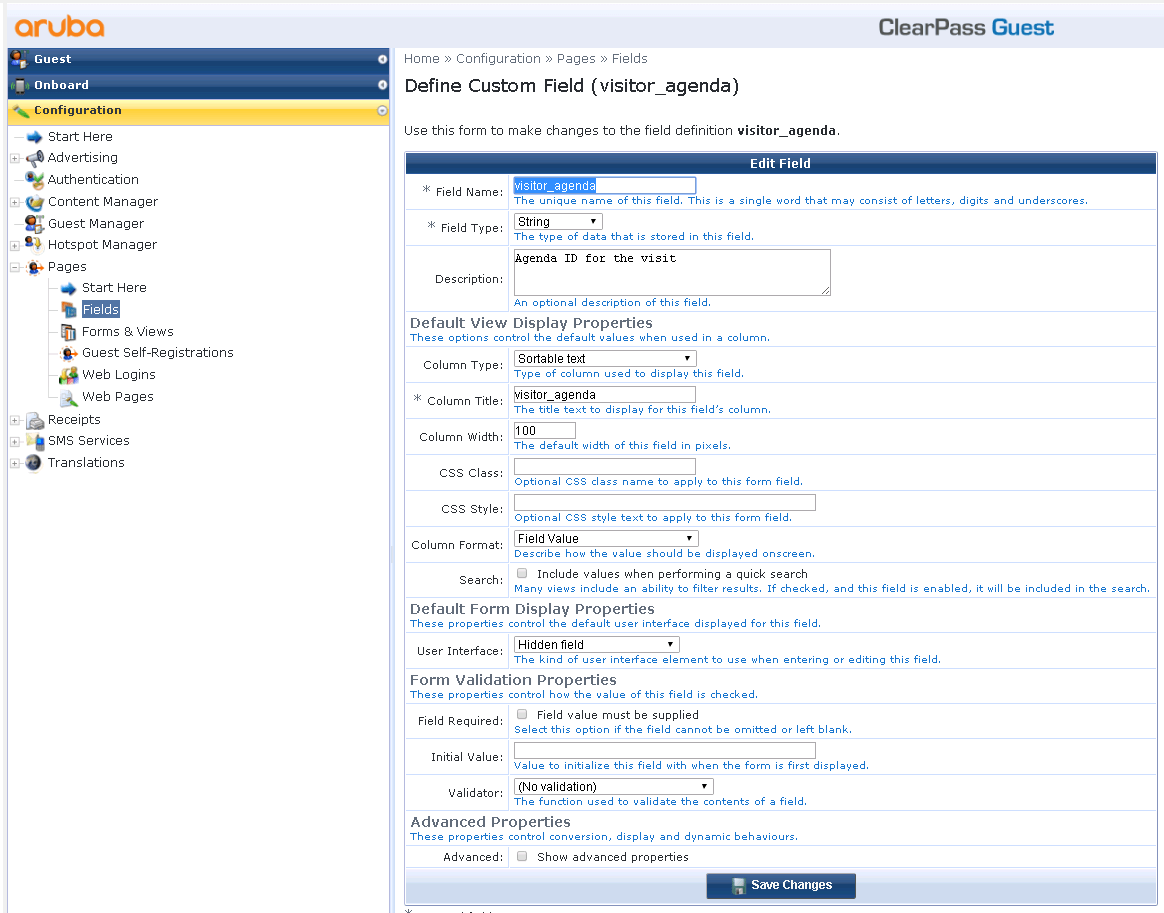The image captures a screenshot of a computer interface. At the top, the word "Aruba" is prominently displayed in orange, lowercase letters. Directly beneath, the words "guest" and "on board" are clearly visible. A rectangular button labeled "configuration" is positioned below these headings.

Further down, the interface is organized into various sections beginning with categories such as "Start Here," "Advertising," "Authentication," "Content Manager," "Guest Manager," "Hotspot Manager," and an indented section labeled "Pages." Within this "Pages" section, subcategories include "Start Here," "Fields, Forms, and Views," "Guest Self-Registrations," "Web Logins," and "Web Pages."

Additionally, there are sections for "Receipts," "SMS Services," and "Translations." At the very top of the interface, the title "ClearPass Guest" is prominently displayed. The word "ClearPass" is formatted with a capital 'C' and 'P,' while the remaining letters are in lowercase. The word "Guest" appears in blue print, contrasting with the black print of "ClearPass."